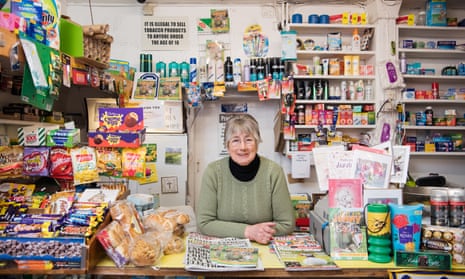The photograph features a woman, approximately 55 years old, standing behind a checkout counter in what appears to be a small convenience or miscellaneous dry goods store. She has glasses, gray hair, and is dressed in a pale green long-sleeve sweater over a black turtleneck. She looks directly at the camera with a smile. In front of her on the counter, various magazines and newspapers are neatly arranged. Surrounding her, the store is stocked with a wide assortment of items: to her left, there are snack cakes, potato chips, candy, and packaged snacks; to her right, jars, glasses, greeting cards, and more candies. Behind her, the shelves are filled with hygiene products like shampoos, conditioners, deodorants, and sunscreens. There's also a variety of household goods, including Bounty paper towels on an upper shelf to the left. The walls, which are white, have additional products hanging on shelves, contributing to the overall impression of a well-stocked, compact retail setting.